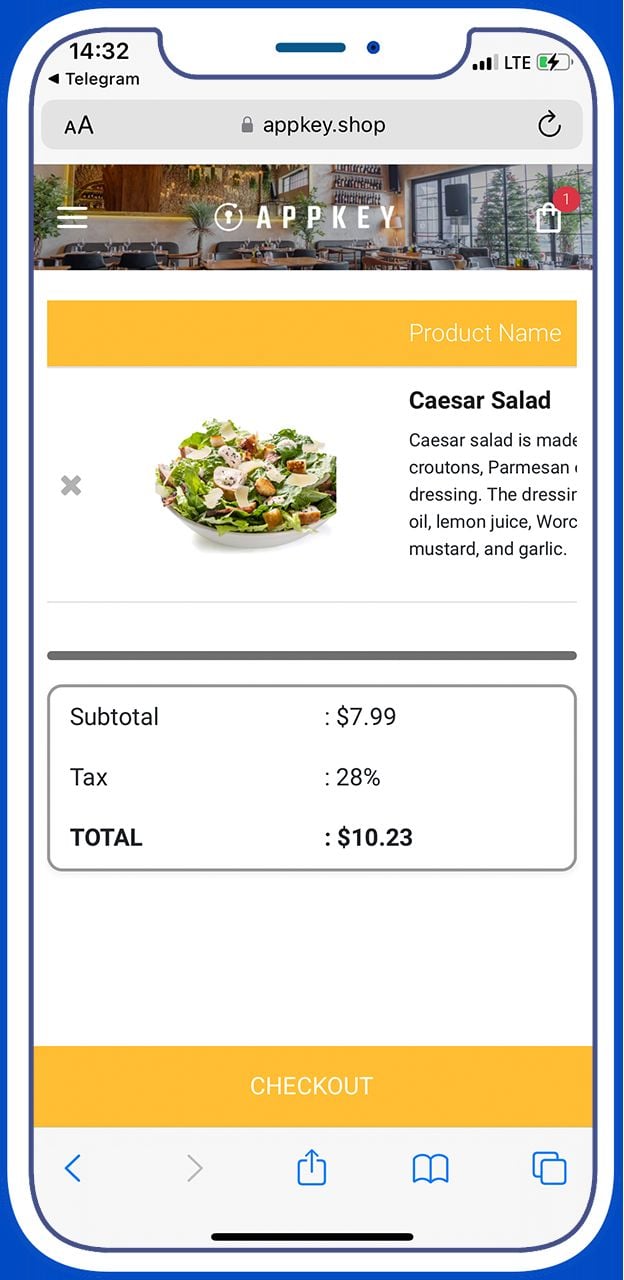The image is a smartphone screenshot displaying several elements. In the upper left corner, the time is shown as 14:32, accompanied by a battery icon indicating approximately 25% charge. Directly beneath the time, there's a Telegram application icon. Below this, a URL bar contains the address "appkey.shop".

The primary content of the screenshot appears to be a webpage from "Appkey," clearly marked in large, white capital letters against the page's background. The page itself presents a room with high tables and tall windows, through which greenery and trees are visible outside. 

In the upper right section of the page, there's an icon resembling a shopping cart, with a red notification bubble displaying the number one. 

Positioned prominently in an orange rectangle is the text "Product Name," beneath which a picture of a Caesar salad is displayed. The description of the Caesar salad includes listed ingredients such as croutons, Parmesan, dressing, oil, lemon juice, mustard, and garlic. However, the full text is partially cut off in the image.

At the bottom of the page, the subtotal for the salad is marked as $7.99.